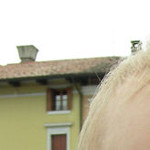The image is a very small, colored photograph taken outdoors during the daytime, featuring a house with a yellowish-green tone. The house has a tall brown roof with a couple of chimneys or vents and a visible guttered downspout running down from the roof towards the house. There is a large window on the second story directly above a red door that is framed in white. The sky is slightly visible in the background. In the lower right-hand corner of the image, there is a partial view of a person with pale skin and pale blonde hair, showing just a corner of their forehead. The details are somewhat blurred and fragmented due to the photograph's small size and zoomed-in nature.